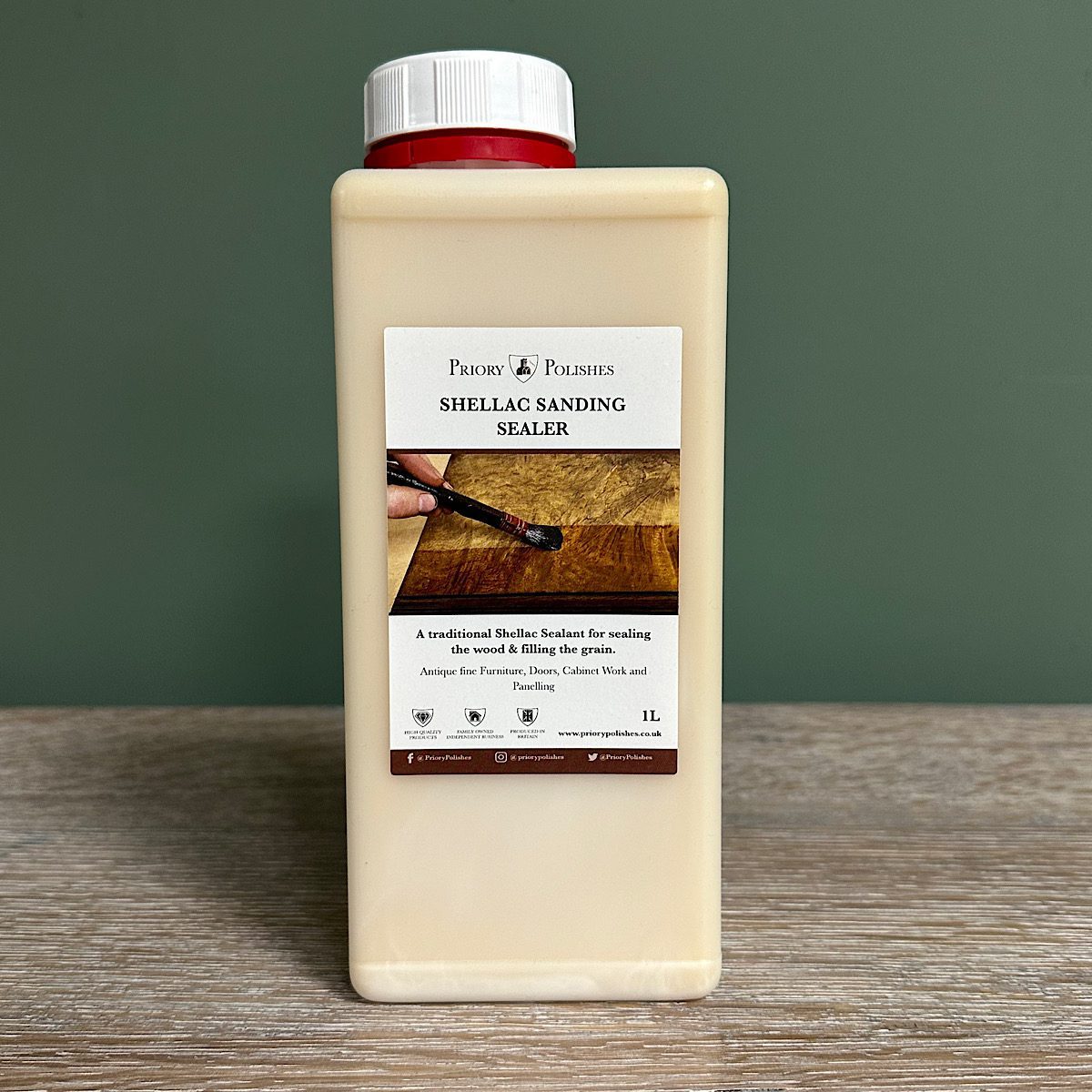The image captures a rectangular plastic bottle sitting on a light wood tabletop, with a green painted wall as the backdrop. The bottle is a light tan color, suggesting it might either be the hue of the plastic or the liquid inside. It is topped with an offset red and white screw cap located on the upper left-hand corner. The bottle features a large, rectangular label on its front. The upper portion of the label has a white background that reads "Priory Polishes Shellac Sanding Sealer." Beneath this text is a photograph of a person using a thin paintbrush to apply the shellac sealer to a piece of wood. The lower part of the label, also on a white background, reads "A Traditional Shellac Sealant for Sealing the Wood and Filling the Grain. Entry Antique Fine Furniture, Doors, Cabinet Work and Paneling." Additionally, the label includes logos and a mention of the website, priorypolishes.com.